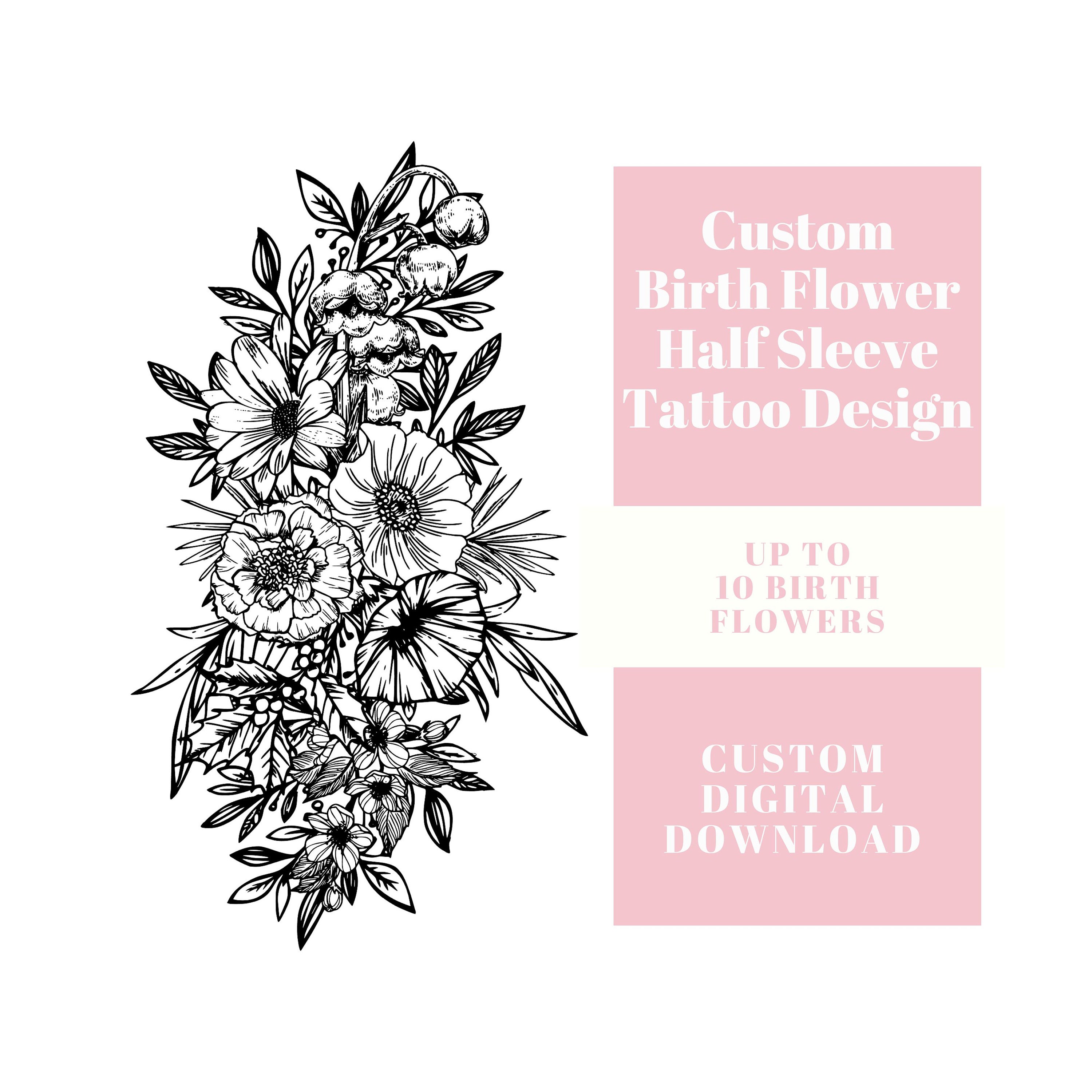This advertisement for tattoo art showcases a beautifully dense, hand-drawn, pen-and-ink floral illustration on the left side, featuring various flowers arranged in a vine-like pattern, with blossoms concentrated in the middle and vines extending above and below. On the right side, three text sections are framed by light pink rectangles. The top pink rectangle contains white text that reads, "Custom Birth Flower Half Sleeve Tattoo Design." Directly underneath, within a white rectangle, pink text announces, "Up to 10 Birth Flowers." The bottom pink rectangle features more white text that states, "Custom Digital Download." The juxtaposition of the detailed floral sketch and the clear, eye-catching text creates a compelling advertisement for custom-designed tattoo services.